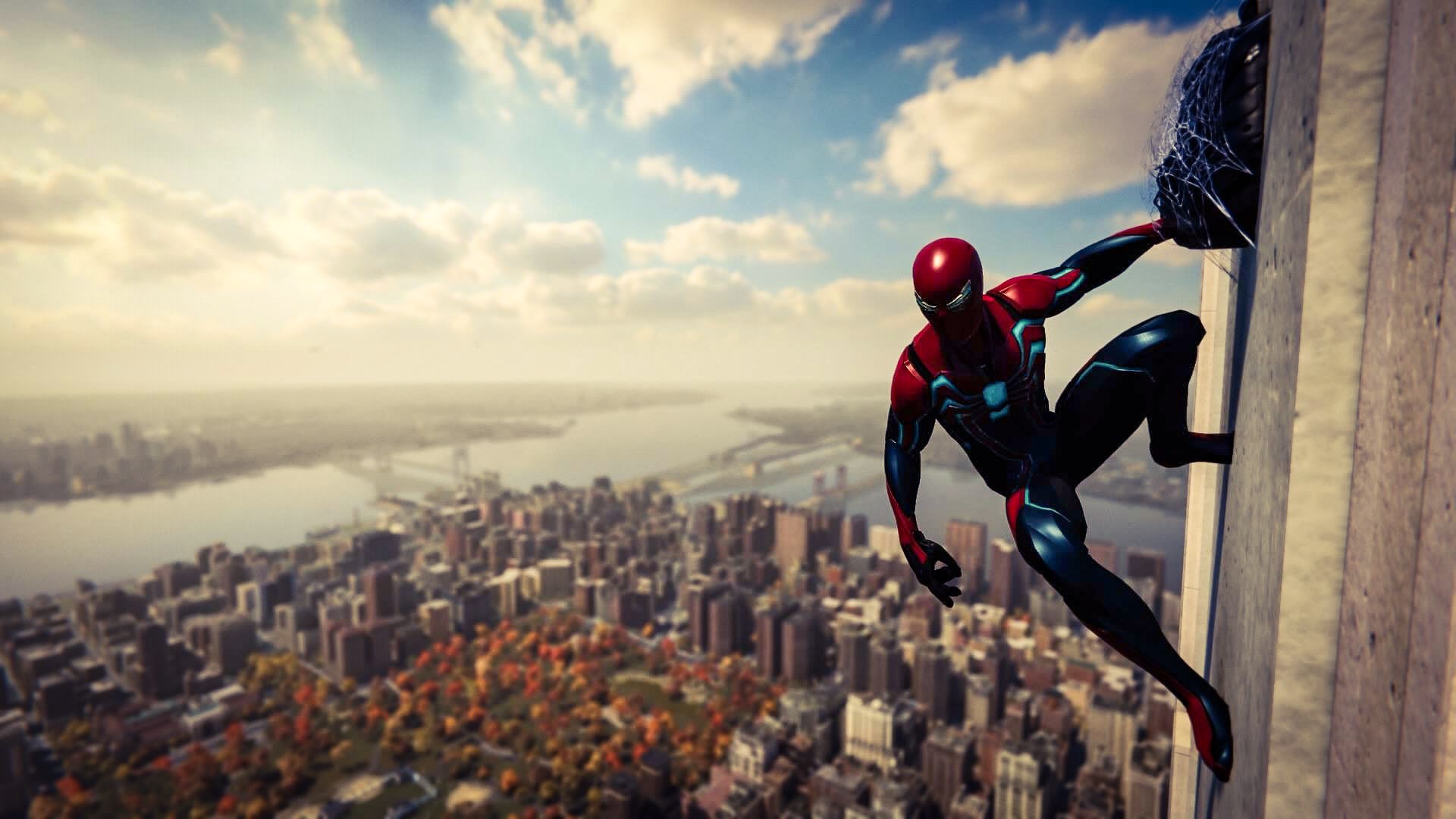In this detailed animated image, we see Spider-Man in a modern-day, shiny, and armored outfit, prominently featuring a light bluish spider emblem on his chest. Spider-Man is perched on the side of a skyscraper, his left leg bent and right leg extended outward, gripping a bunched-up spider web with his left hand. The perspective is from the top of an extremely tall building, overlooking a cityscape with numerous high-rise buildings and a body of water with a suspension bridge. The sky above is a vibrant blue, dotted with fluffy white and grey-centered clouds. The backdrop of the city, which includes some orange and red-hued trees suggesting a fall setting, is softly blurred, emphasizing Spider-Man as the focal point. Despite the slightly dark and blurry quality of the image, which might be a photograph of an animated scene from a computer game, the right side of the frame captures a well-focused close-up of the skyscraper and Spider-Man in his dynamic pose, ready to leap into action.